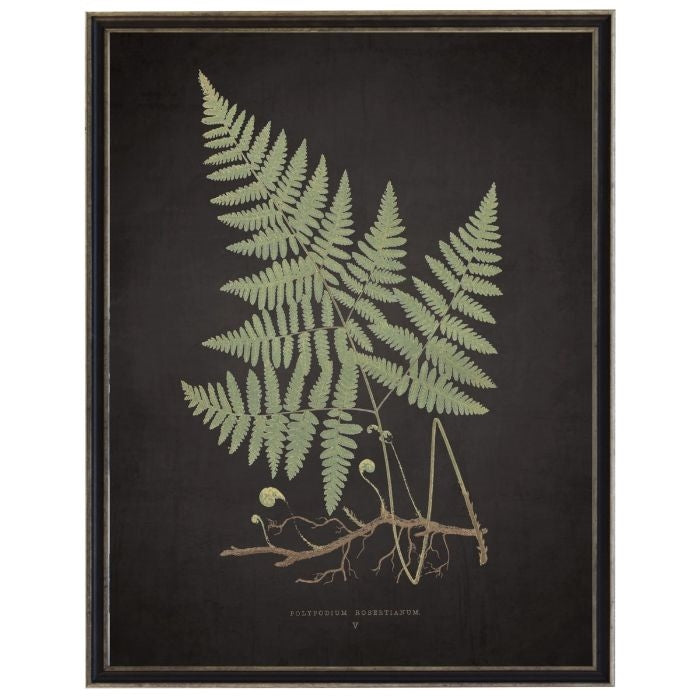The image is a detailed photograph, not a painting, of a framed botanical print displayed on a wall. The frame is black with lighter gray edges, and it encloses a striking black background that enhances the simplicity of the artwork. The main subject of the photograph is a fern, more specifically identified as "Polypodium Robertianum IV," based on the elegant text inscribed at the bottom of the print. The fern features light, muted green leaves, almost resembling a sage color, and is arranged with larger stems at the bottom tapering to smaller ones at the top, forming a pyramid or Christmas tree-like shape. The fern’s roots are exposed, adding to the botanical accuracy and charm of the piece. The natural simplicity and muted color palette make the image look like a refined print likely used for aesthetic or educational purposes.